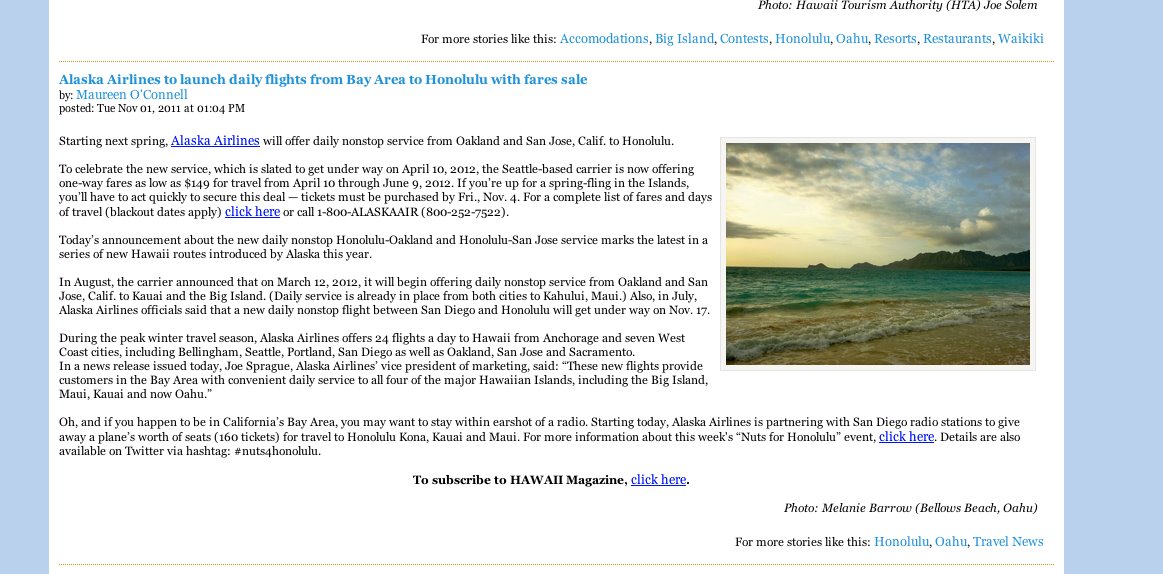Screenshot of a promotional graphic on a blue background with white text at the center. The image credits "Hawaii Tourism Authority (HTA) / Joe Salem." The text reads: "For more stories like this, visit Accommodations Big Island Contest." 

Below it, in bold, is "Honolulu, Hawaii." 

The graphic also mentions various resorts and restaurants in the Waikiki area. 

A small picture within the graphic depicts a beach scene. 

At the bottom, it's announced that Alaska Airlines will launch daily nonstop flights from the Bay Area, specifically Oakland and San Jose, California, to Honolulu, starting next spring. This information was posted by Marine O'Connell on Tuesday, November 1, 2011, at 1:04 PM.